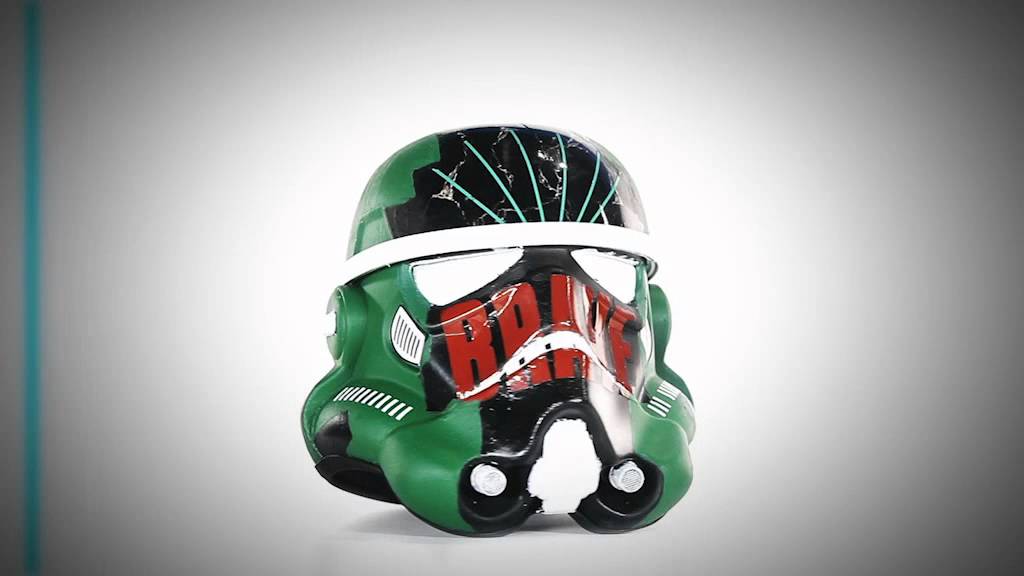The image depicts a horizontally rectangular scene featuring a distinctively painted Star Wars Stormtrooper helmet. Set against a gradient gray background that brightens towards the center due to artificial lighting, the helmet stands out with its vibrant and unconventional color scheme. A vertical blue line runs from top to bottom just to the left of the center, adding an additional visual element.

The helmet, traditionally white, has been creatively repainted green. The upper section, particularly the forehead, is marked by a black area adorned with neon green vertical lines. The visor conveys an intense look with its stark white hue, contrasting sharply with the altered color palette. Below the eye section, at the nose, the helmet features a black band inscribed with the word "BRAKE" in red text, though some interpretations suggest it might also read as "BAKE" or "BRAVE."

Interestingly, the helmet carries signs of wear and damage, adding to its unique character. The overall image is meticulously detailed, highlighting the imaginative rendition of an iconic piece from the Star Wars universe.